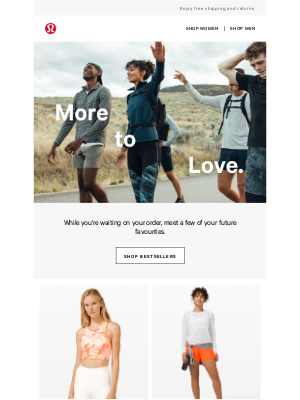The image, sourced from a website, is set against a white backdrop. In the upper left corner, there is a red circle featuring a white horseshoe-like shape inside it. In the upper right-hand corner, although the black text is blurry and unreadable, below it, clearly written in black, are the words "Shop Women" followed by a line and then "Shop Men." Below this text, the primary image shows five people walking along a road with a field or possibly a desert with brush in the background.

On the left-hand side, a black gentleman is dressed in a gray long-sleeve zip-up shirt paired with shorts. Next to him, a black woman, her hair pulled back in a ponytail, is wearing a blue long-sleeve shirt and black leggings that feature a blue, white, and black pattern from the thigh down. Behind her, a partial view of an arm in a white long-sleeve shirt and black shorts, appearing to belong to a Caucasian person, is barely visible. To their right, a Caucasian man is dressed in a white long-sleeve shirt and black shorts, with a black backpack. On the far right, partially cut off, is another Caucasian man with short brown hair, lifting his hand to the back of his head. He is seen wearing a black t-shirt and gray shorts.

Across the image, white text overlays various parts of the figures. On the chest of the black man on the right, it reads "more," across the waist of the black woman, it says "two," and in front of the Caucasian man with the backpack, it says "love." Below the main image, black text states, "while you're waiting on your orders, meet a few of your future favorites," followed by a white box with the black text, "shop best sellers."

Beneath this text box are two additional pictures. The one on the left features a blonde Caucasian girl wearing a peach and white crop tank top and white pants. The image on the right showcases a light-skinned black woman with her hair pulled back, dressed in a long-sleeve white shirt and a pair of gray shorts that have a neon orange front.